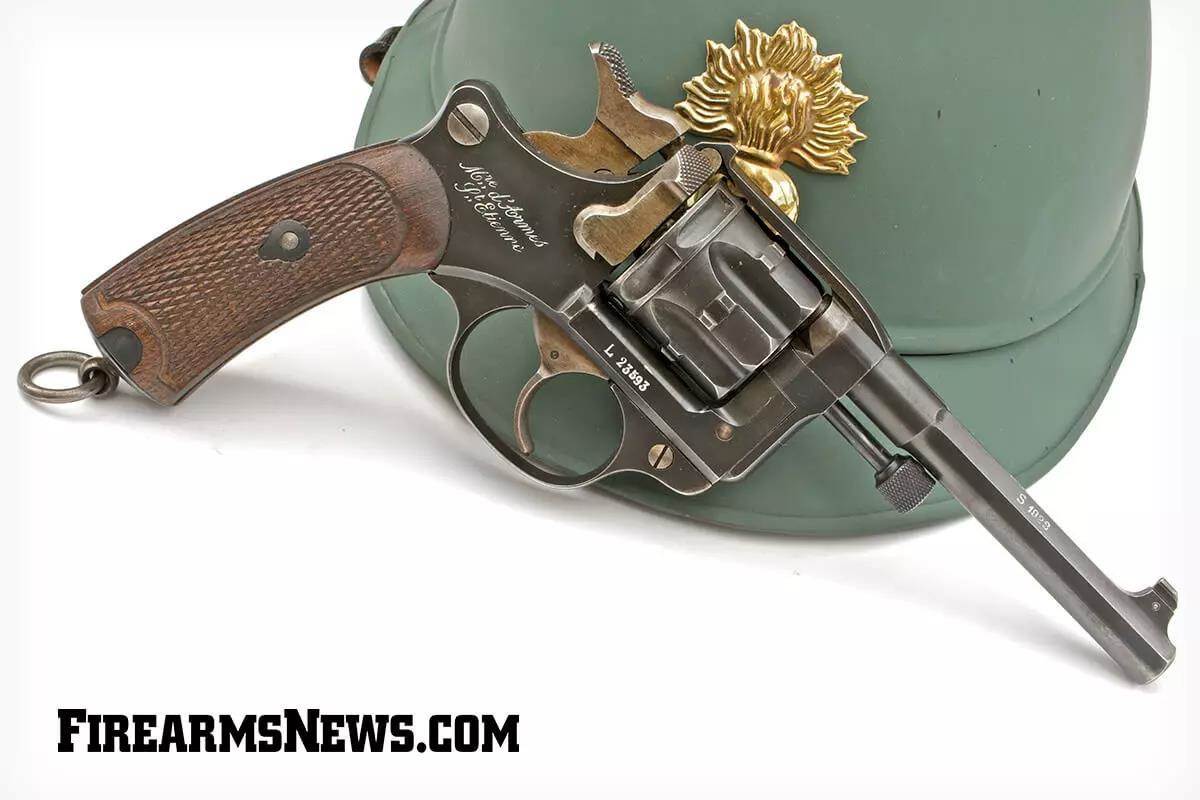The image on a white background showcases a vintage-looking revolver placed in the foreground. The revolver features a burnished brown body with a wooden grip that shows signs of wear, indicating its age, yet remains well-maintained. The trigger exhibits a coppery hue, and the barrel and chambers, though slightly rusty, retain a dark gray color. A silver metal ring hangs off the end of the handle, adding to its worn charm. Positioned behind the revolver is a soft green, army-type helmet adorned with a highly polished, reflective golden badge resembling a sun-like star. The helmet and revolver sit on a white tabletop. In the bottom left corner of the image, the watermark "firearmsnews.com" is clearly visible.